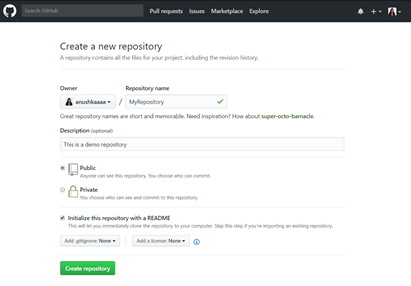The image depicts a user interface for creating a new repository on a version control platform, possibly GitHub. The central focus is on a form used to set up the repository. The interface includes several key components:

1. **Repository Settings**:
   - The repository name field is visible, intended for the user to input the name of the repository.
   - The form highlights an area indicating it is a "demo repository."
   - There is a selection option between "Public" and "Private" repositories, with "Public" being currently selected. This choice dictates the visibility of the repository to other users.

2. **Initialization Options**:
   - A checkbox option labeled "Initialize this repository with a README" is present, with "README" capitalized; the checkbox is marked, indicating that the repository will include an initial README file.

3. **Action Button**:
   - At the bottom of the form, there is a prominent green button labeled "Create repository," which users would click to finalize the creation process.

4. **Interface Layout**:
   - The overall interface features a clean, white background that enhances readability.
   - At the very top of the interface, a navigation bar includes small-text options like "Marketplace" and "Explore," although they are slightly hard to read.

5. **Owner Information**:
   - A section highlights the repository owner within a square overlay, providing clarity on who manages the repository.

6. **User Icon**:
   - In the top-right corner, there is a small user profile image or icon, likely representing the person creating the repository.

7. **Pull Requests**:
   - The "Pull requests" tab is highlighted, suggesting focus or recent activity in that section.

The image effectively guides a user through the process of creating a new repository, specifying its visibility, initializing it with a README file, and completing the setup with the "Create repository" button.